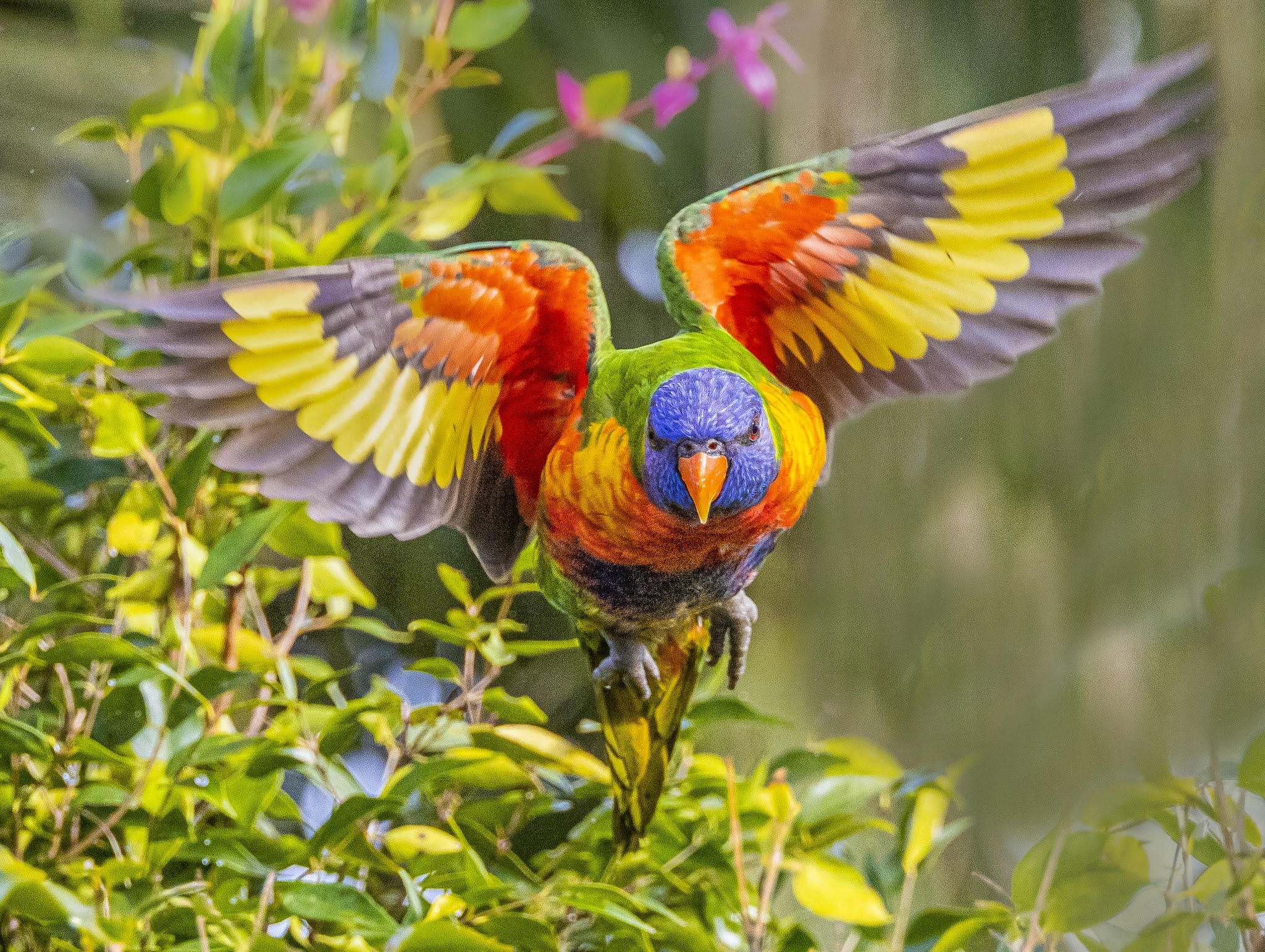This photograph captures a vibrant parrot in the midst of taking flight, seemingly poised to push off from a perch adorned with small, delicate pink flowers. The parrot's wings are dramatically pulled back, showcasing an array of striking colors: green, orange, and gray, with yellow feathers interspersed, all outlined with streaks of black. Its back is primarily green, while its belly displays a dynamic blend of orange, red, yellow, and some darker shades possibly hinting at blues. The bird's bright blue head and red eyes sharply contrast with its orangey beak, adding to its striking appearance. Its legs are gray, tucked behind its body as it faces the camera, caught mid-motion. The backdrop is softly blurred, highlighting a leafy tree and a hint of a fence, ensuring the focus remains on the parrot’s vivid plumage and poised stance.